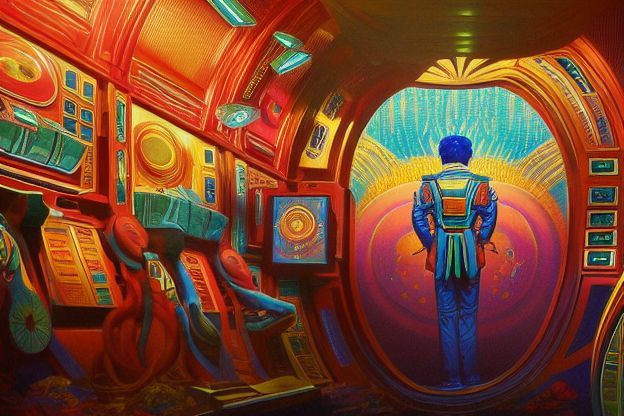The image appears to be a vibrant, technicolor painting or a comic book-style illustration, characterized by its vivid, eye-catching colors. Dominated by fiery oranges, reds, and yellows, the scene is filled with additional hues like turquoise, deep purple, indigo, and hot pinks. It depicts a man with indigo blue hair, dressed in a flashy, space-themed outfit reminiscent of an astronaut or a spaceship captain's uniform that combines elements of orange, red, yellow, blue, and green. He stands with his back to the observer, gazing out of a round doorway in what seems to be a spaceship. Surrounding him are numerous screens, buttons, displays, and control panels, contributing to the futuristic atmosphere. On one side, there appears to be a gaming station complete with a chair, adding to the abstract, sci-fi aesthetic of the scene. The overall composition portrays a colorful and dynamic environment, merging elements of space travel, technology, and surreal artistry.